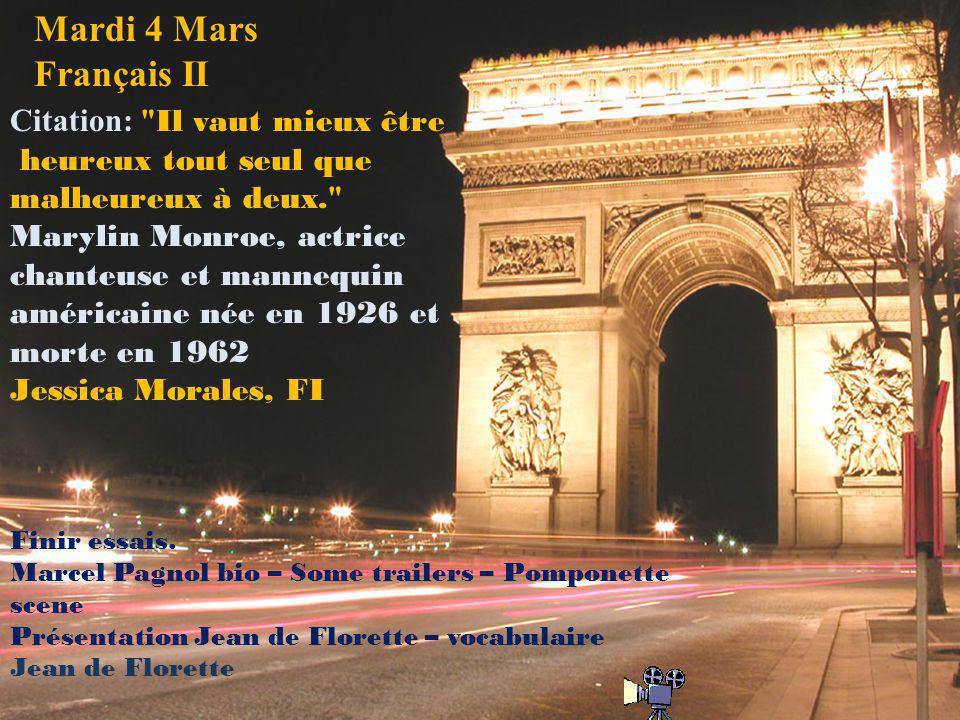The image is a captivating nighttime color photograph of the iconic Arc de Triomphe in Paris. The large, illuminated stone archway stands prominently on the right side of the frame, set against a dark background. The foreground features the dramatic trails of taillights from passing cars and a row of glowing streetlights, painting a lively picture of Parisian nightlife.

On the left side of the image, there's French text at the top that reads "Mardi for Mars Français II" in a mix of white and yellow letters. Further down, beneath this, the text mentions Marilyn Monroe, detailing her as an American actress born in 1926 and passing in 1962. Additionally, the name Jessica Morales, F.I., appears, and there is more French text in blue at the bottom left of the image, possibly crediting the creators.

Near the center, slightly to the right, there is a cartoon depiction of a movie camera, adding an artistic touch to the scene.